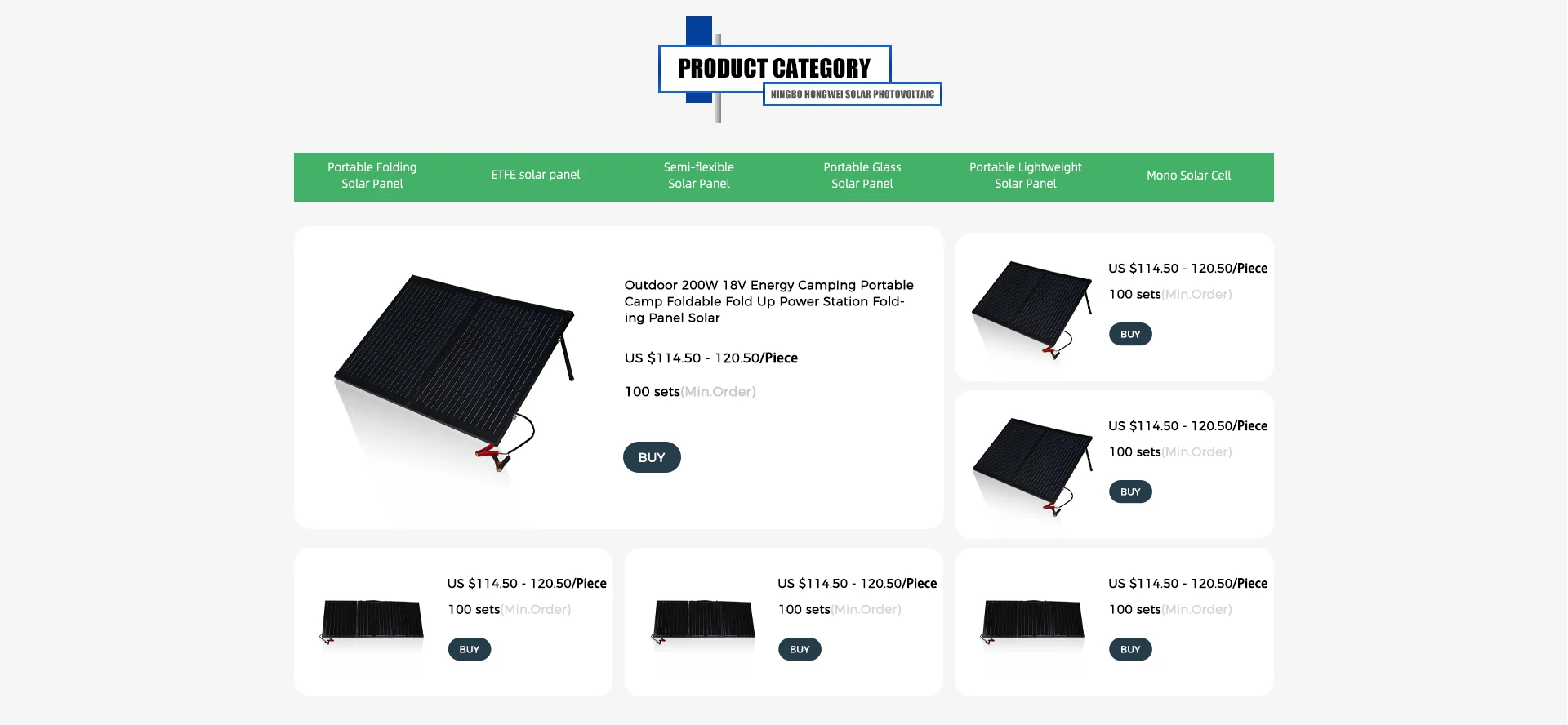The image features a rectangular layout with its horizontal orientation spanning from left to right against an off-white or gray background. At the top center of the image, the text "Product Category" is prominently displayed within a blue-bordered box. Slightly below and to the right of this, there is another outlined box, though the text within it is difficult to discern due to its small print.

Beneath these titles, a green border encloses white text, which is similarly challenging to read, presumably describing "Portable Folding Solar Panels." Further down, the main section of the image is divided into six segments or sections, each featuring a black rectangular image representing the solar panels.

Accompanied by text, these sections detail: "Outdoor 200 Watt 18 Volt Energy Camping Portable Camp Foldable Fold-Up Power Station Folding Panel Solar." The pricing for these solar panels is listed as $114.50 each, with an option of $120.50 per piece for 100 sets. Positioned next to the pricing information is a black oblong button with the word "Buy" written on it.

Surrounding the central image are five smaller images, each resembling the larger rectangular depiction of the solar panels, illustrating various aspects or configurations of the product.